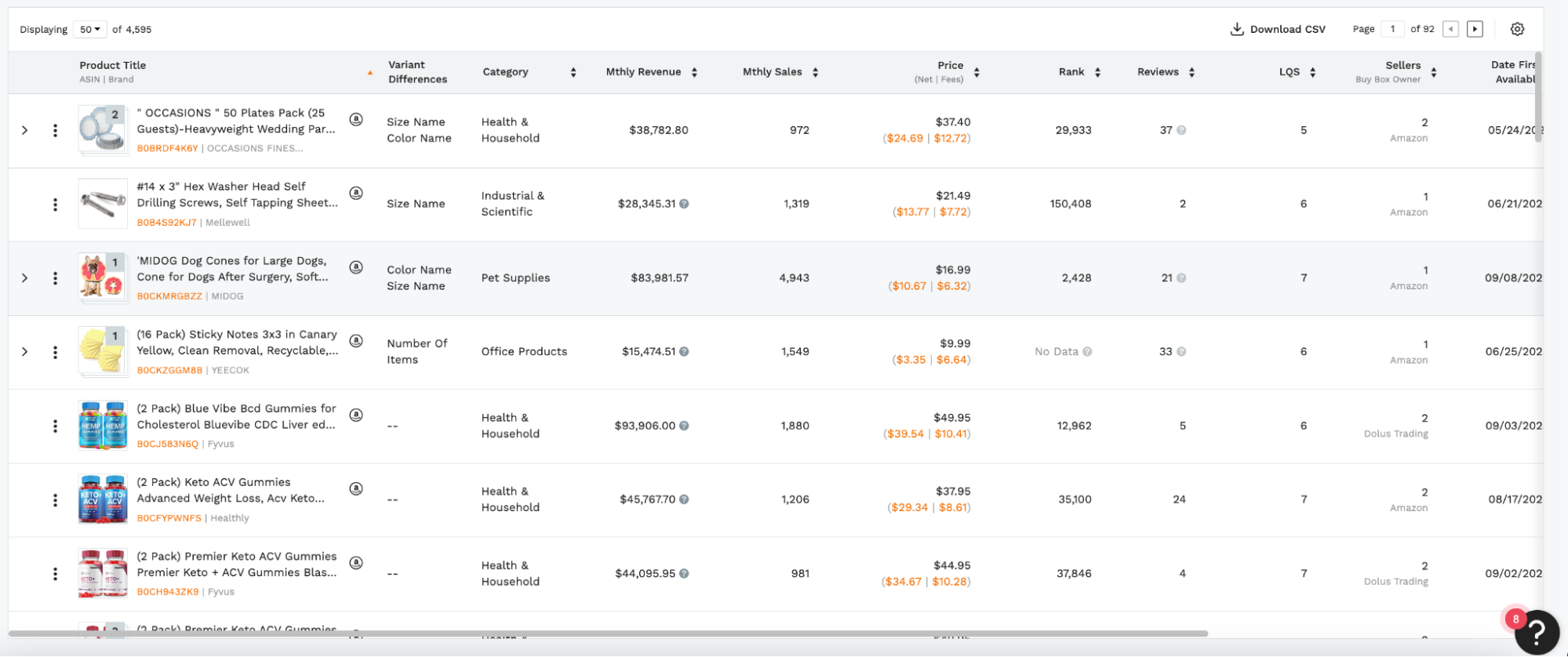This image is a detailed screenshot taken from a laptop display in landscape mode. It captures a data management interface displaying sales information. In the upper left-hand corner, there is a text showing "Displaying 50 of 4595," indicating the number of entries currently viewed. The upper right-hand corner displays options to "Download CSV" and navigational elements labeled "Page 1 of 92" along with back and forward buttons.

The interface lists multiple rows and columns under various sortable tabs including: Product Title, Variant, Differences, Category, Monthly Revenue, Monthly Sales (abbreviated), Price, Rank, Reviews, LQS (a quality score), Sellers, and Date First Available. Each row within this table contains products along with their specific details and images on the left.

Here are some examples of product entries listed:

1. **Occasions 50 Plate Pack** - includes an image on the left.
2. **14 x 3 Hex Washer Head Self-Drilling Screws** - includes an image on the left.
3. **My Dog Dog Cones for Large Dogs** - includes an image on the left.
4. **16 Pack Sticky Notes 3x3 in Canary Yellow** - includes an image on the left.
5. **2 Pack Blue Vibe BCD Gummies for Cholesterol** - includes an image on the left.
6. **2 Pack Keto ACV Gummies Advanced Weight Loss** - includes an image on the left.
7. **2 Pack Premier Keto ACV Gummies** - includes an image on the left.

Each row appears to include additional columns with detailed descriptions such as Size, Name, Category (like health and household), Monthly Revenue, suggesting that this table is a comprehensive breakdown of product performance. This screenshot likely represents someone’s detailed sales data, illustrating their profits and product statistics.